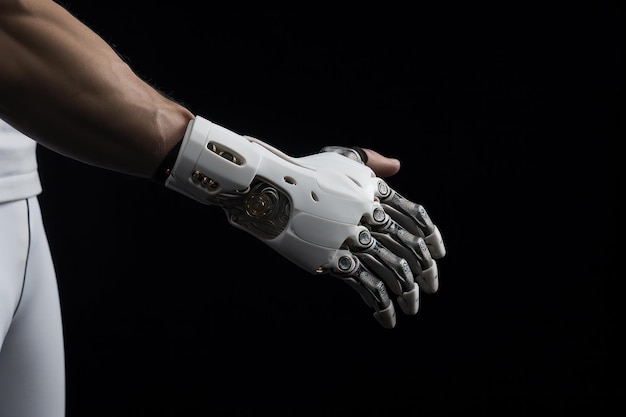In this detailed photograph, a man's muscular, veiny forearm extends from the upper left corner of the image, culminating in a sophisticated, off-white to light gray bionic hand with intricate dark gray joints and robotic fingers. Only his natural thumb remains exposed, seamlessly blending into the meticulously designed prosthetic. This high-tech device features distinctive components, including silver-like dark gray fingers that taper into light gray, presumably rubberized, fingertips for tactile function or touchscreen use. Near the wrist, there are visible sections with internal wiring and gadgetry, offering a glimpse into the mechanical sophistication that enables the hand to mimic natural movements. The man's attire consists of white-grayish pants and a similarly colored shirt, contrasting sharply against the predominantly black, stark background, which accentuates the detailed craftsmanship of the bionic hand.